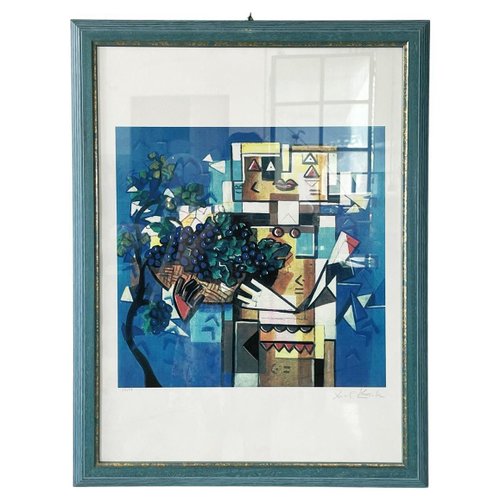We're looking at a photograph of a framed, abstract painting set against a plain white background with no visible borders. The rectangular frame, about an inch and a half to two inches wide and three inches high, is light blue with a gold inset. The picture inside has a white border that is thicker at the top and bottom. The painting is a geometric depiction of a person, featuring yellow rectangles for the head and body. The person has triangle-shaped eyes, red triangle blushed cheeks, a pair of lips, and a white square for the neck. One arm is composed of white, black, and red triangles. The figure is holding a brown basket containing either blueberries or grapes with green leaves. To the left of the figure, there is a black tree with green leaves and more berries hanging. The image is covered with glass, which reflects the surrounding environment. The reflection reveals a window with six grid panes to the upper right and the top of the photographer's head in the center. To the left of the reflection, there appears to be a door. The painting also includes abstract elements like diamond shapes, distorted hands, and pillars, adding to its puzzling and intricate nature.